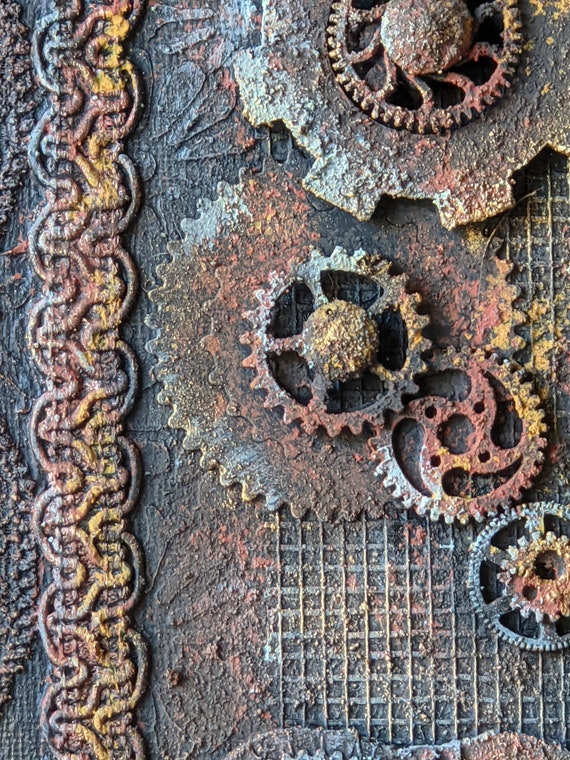This detailed image presents a textured and rusted metallic setting, appearing as an artful painting or photograph, focused on the mechanical theme of gears and cogs. Dominating the upper right corner is a large gear with pronounced sprockets and a smaller central gear, both exhibiting signs of wear and rust. Directly below, another substantial gear of similar size features finer sprockets, while two intermeshing gears are visually distinctive; one has a smooth, round center, and the other a wavy central design punctuated with small holes. The latter engages with a smaller, blue and orange gear situated at the bottom right. A decorative, chain-like element runs vertically on the image's left side, complementing a series of wavy lines beneath. The background integrates a grid-like, waffle pattern, emulating the look of graph paper, overlaid with the impression of mildew and growth in hues of blue, yellow, and red. The gears, primarily gray and brown, suggest a narrative of time and decay, underscored by the careful depiction of rust and textured surfaces throughout the artwork.